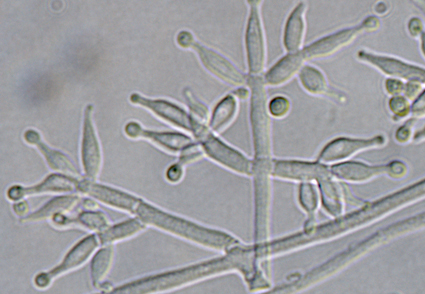The image depicts microscopic bacteria or cells observed through a microscope. These cells have a distinct shape, characterized by rod-like structures adorned with green spherical formations at their tips. The rods, which vary in length and orientation, include some that extend diagonally from the bottom right to the upper left. The background is predominantly gray, featuring two shadowy or faded circular spots in the upper left corner. The overall scene resembles a network of connected branches or stems with leaves, where each "leaf" is a circular shape of varying sizes, contributing to a slightly greenish hue. The arrangement and fine details give the impression of intricate, organic patterns set against a stark gray backdrop.